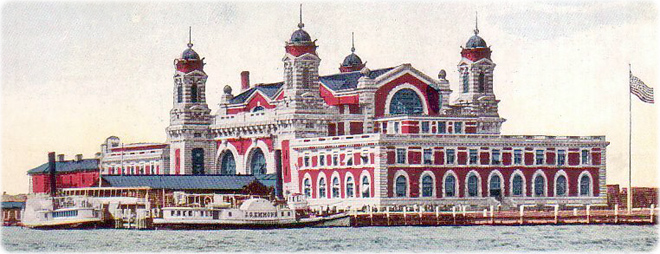The painting depicts a grandiose, older colonial-style building set against a water body, possibly a river or seaport in the United States, exuding a patriotic essence evident by the American flag fluttering on a flagpole to the right. The architectural marvel, characterized by its red and white brick or stone construction, features multiple arches, white columns, and glass windows, with blue accents highlighting the roof and windows. The building is adorned with four prominent gold- or metal-tipped spires that lend a Gothic cathedral-like appearance. In the foreground, two or three white riverboats, reminiscent of steamboats, are docked at a pier with a blue-roofed covering extending over the water. The scene is set under a hazy, creamish gray sky, enhancing the nostalgic and serene atmosphere of this port-side location.